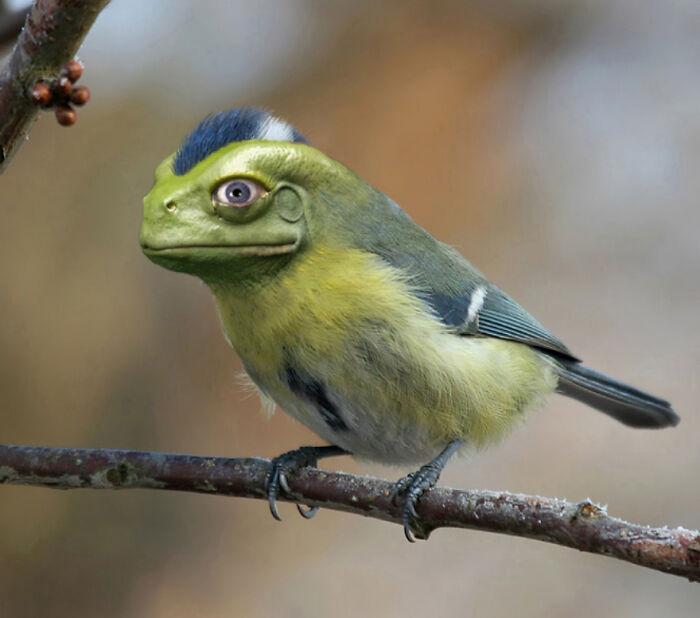This computer-generated image features a peculiar bird-like creature with a reptilian twist. Standing upright on a thin, horizontal brown tree branch with its black claws wrapped firmly around it, the creature dominates the center of the square image. Its head is a green, frog-like face with slick skin, complete with white eyes, large blue irises, and black pupils. A striking, spiky mohawk of blue and white hairs runs down the center of its head. The creature's mouth, shaped more like that of a frog, is closed.

The body retains avian characteristics, with bluish-green and gray-blue feathers adorning its back and a long tail extending behind it. The belly is covered in yellow fuzz with a prominent black streak running through the white underbelly. The setting appears outdoors, characterized by a blurred backdrop of gray and brown hues, conveying a sense of depth but lacking distinct details. In the upper left corner, another tree branch with berries peeks into the frame. The overall image blends natural elements with imaginative, fantasy-like alterations.